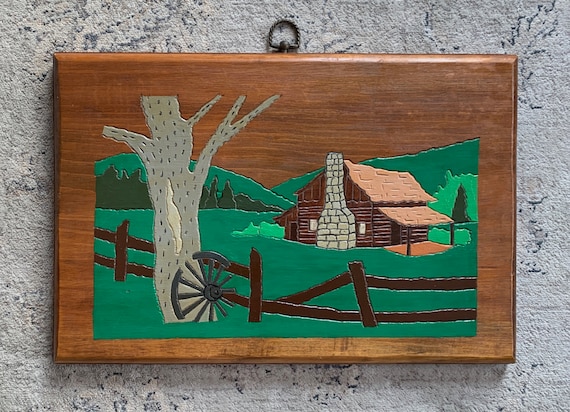This photograph captures a detailed wooden art piece hanging on a gray cement wall. The piece itself is a rectangular dark brown plaque with a beveled edge and a small metal loop at the top for hanging. The scene carved and painted onto the wood depicts a rustic countryside. 

In the foreground, a weathered wooden fence stretches across the entire scene, interrupted by a broken section. A large gray tree, devoid of leaves, anchors the scene with an old wagon wheel leaning against its base. The grass and rolling hills are rendered in medium to dark green hues, with the hills forming a V-shaped valley in the middle of the picture. 

To the right, the focus turns to a quaint log cabin, characterized by its dark brown logs, gray stone chimney, beige roof, and covered porch. Beside the cabin stands an evergreen tree, painted in a darker shade of green to contrast the lighter greens of the hills. The sky above remains the natural color of the wood, unpainted, adding to the rustic charm. The entire piece combines both carved and painted elements, giving it a textured, almost puzzle-like appearance.